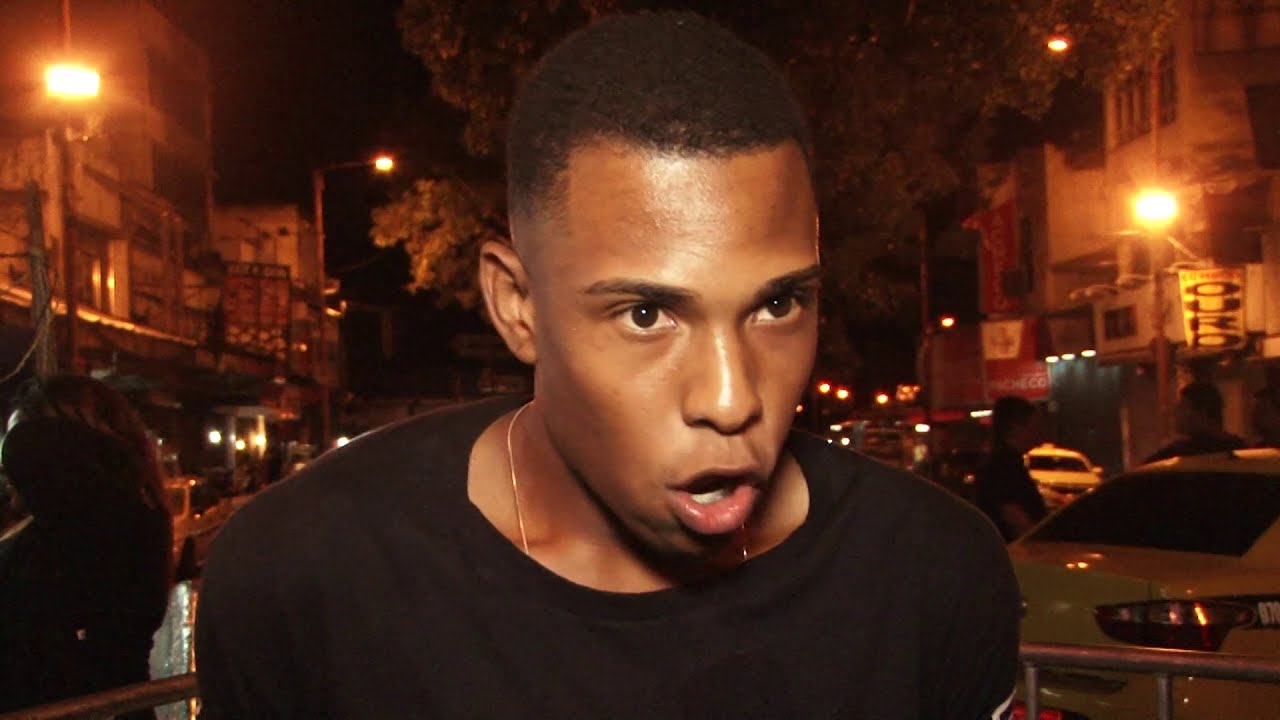The photograph captures a young black man in his 20s, standing outdoors in an urban setting at night. The image is in landscape view and shows him from the shoulders up, with a close-up focus on his face. He has brown skin, very short black hair, and dark brown eyes. He is wearing a black t-shirt with a thin gold or silver chain peeking out from the neckline. His mouth is open in an 'O' shape, suggesting he is either speaking with enthusiasm or yelling, which reveals his teeth. The background displays a bustling city scene, crowded with people, cars, and street lights. Buildings and signage frame each side of the image, while a tree stands in the middle of the street behind him. The sky is pitch-dark, emphasizing the night-time setting.